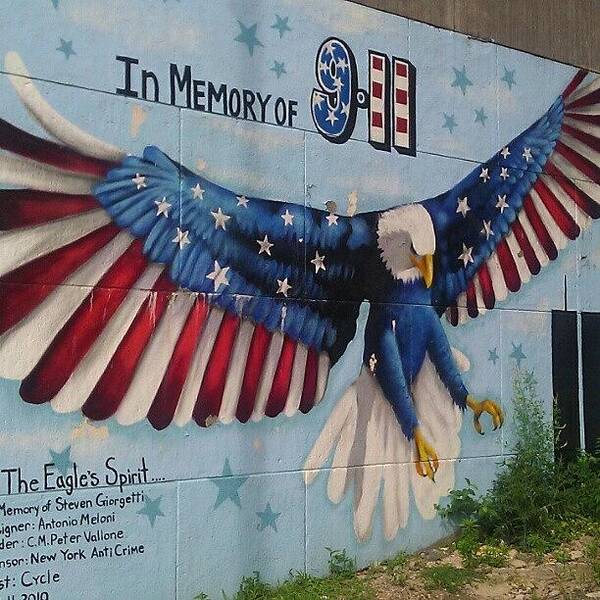This image features a richly detailed mural painted on the side of a building, dedicated to the memory of 9/11. The mural's centerpiece is a magnificent American bald eagle, its wings dramatically spread wide, giving the illusion of it swooping downward. The eagle's body and upper wings are adorned in a vivid blue with white stars, mirroring the American flag, while its extended feathers transition into striking red and white stripes. The eagle's head is white, complete with a yellow beak, and its talons are also yellow. Below, the tail feathers are purely white. The mural's background is a soft light blue, interspersed with faint greenish-blue stars, enhancing the patriotic theme.

At the top of the mural, the words "In Memory of 9-11" are prominently displayed. The '9' is depicted in blue with white stars, and the '11' is designed to resemble the Twin Towers, featuring red and white stripes. In the bottom left corner, the mural bears the text "The Eagle's Spirit, in memory of Stephen Giorgetti" along with the names of the designer, Antonio Maloney, C.M. Peter Vallone, and the New York Anti-Crime Cycle. This detailed and evocative artwork serves as a poignant tribute to those affected by the events of September 11.